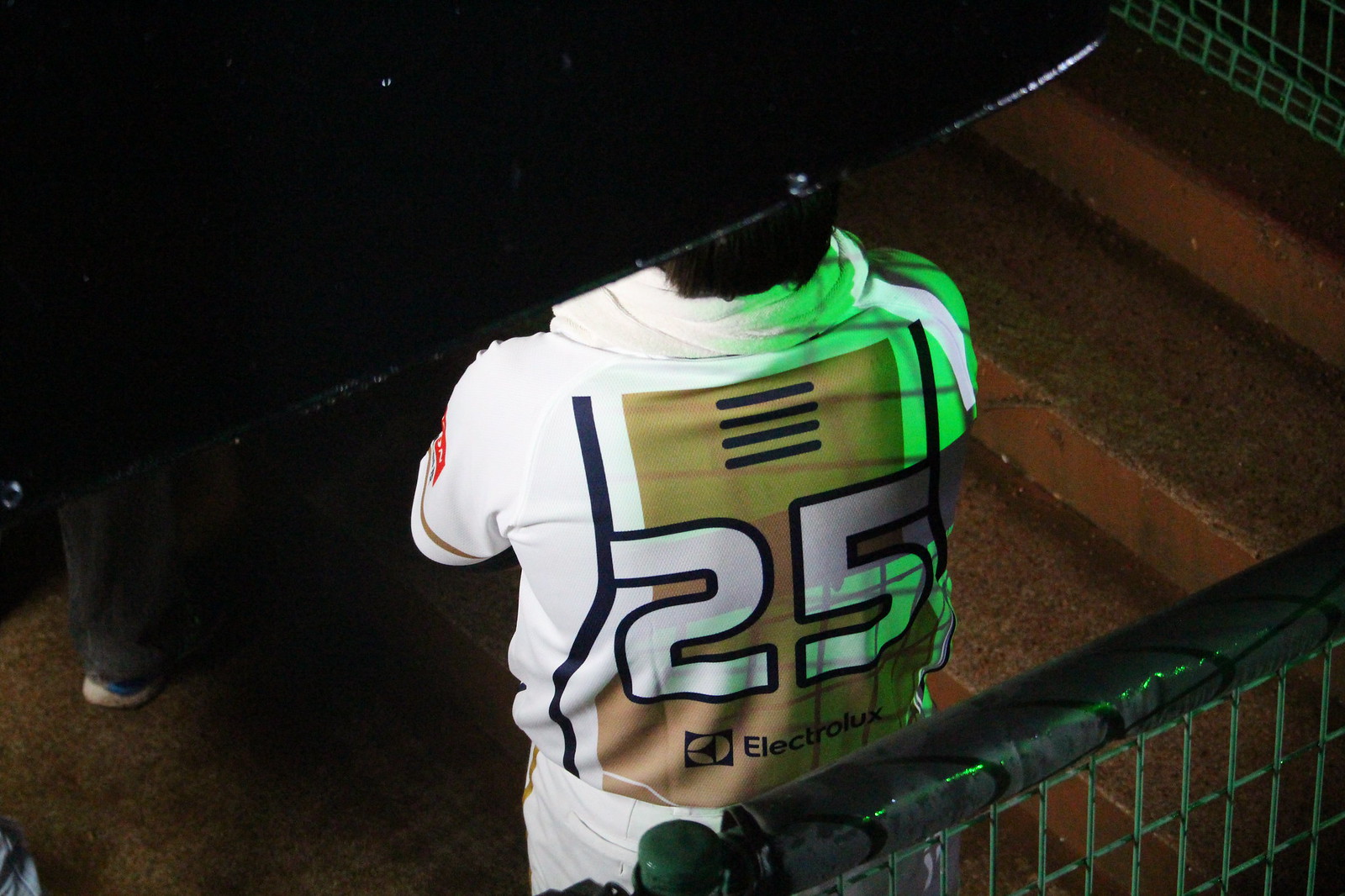In this nighttime color photograph, a person is centered in the image, with their back turned to the camera. The individual is wearing a white jersey that prominently features a logo for the company Electrolux, alongside the number 25, which is white with a black border and a gold backing. The jersey also contains accents of tan, blue, red, and black. The person's arms are crossed in front of them, and their dark-colored hair is partially visible. A bright green light illuminates their right shoulder. To the right of the person are some concrete steps, and a black metal grate fence extends diagonally to the top right of the image. In the bottom left corner, a leg with a blue and white shoe is visible, indicating the presence of another person. The overall scene is dimly lit, reinforcing the nighttime setting.